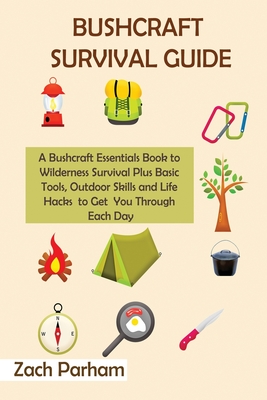This image features the cover of a bushcraft survival guide authored by Zach Parham, showcasing an array of detailed illustrations of camping and outdoor essentials. The title "BUSHCRAFT SURVIVAL GUIDE" is prominently displayed in dark brown, all-caps lettering at the top of the cream-colored cover. Below the title, an olive green text box with dark brown lettering reads, "A bushcraft essentials book to wilderness survival, plus basic tools, outdoor skills, and life hacks to get you through each day." Scattered across the cover are vivid illustrations including a red lantern with a flame, a green and yellow camping backpack, pink and green carabiners, a leafy tree, a metal kettle, a green pitched tent, a log campfire, a compass, a frying pan with bacon and an egg, and a red-handled knife. The author's name, "Zach Parham," is inscribed in a white box with brown letters at the bottom left corner. The background of the image is a beige-pink hue, adding a warm tone to the overall design.